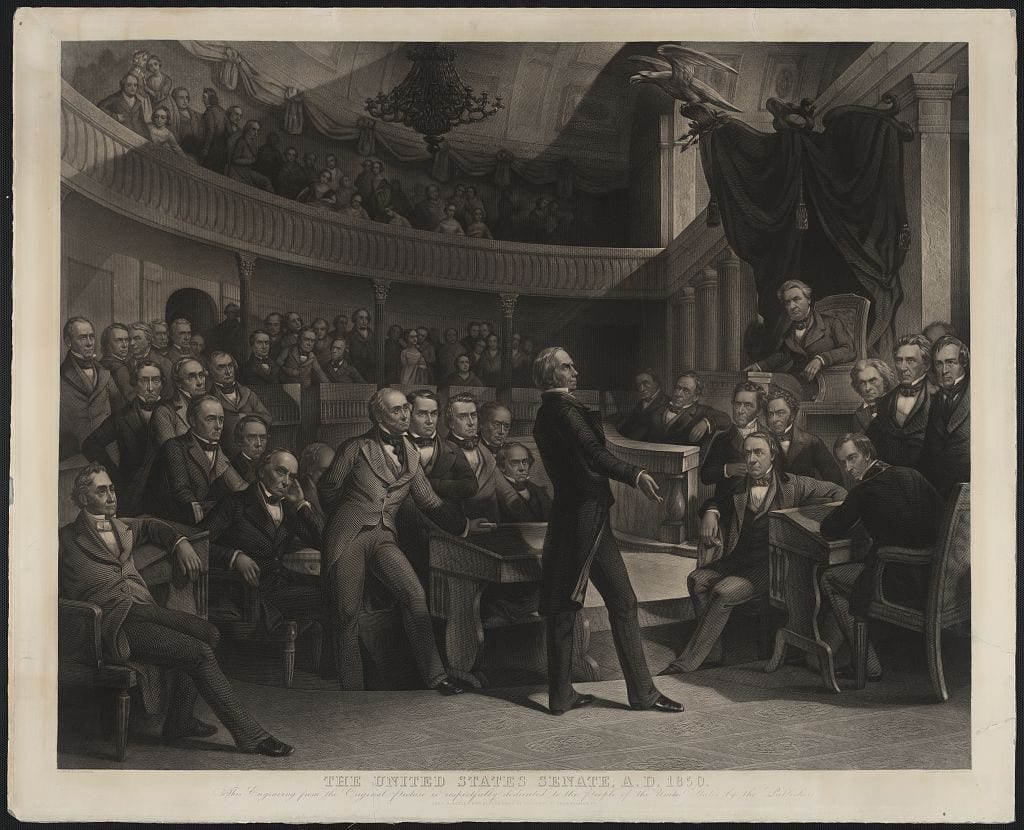This is a detailed drawing, rendered in black and white on parchment with a white border, depicting the United States Senate chamber in 1850. The image centers around a man in a suit, who stands as the focal point, slightly leaning back and dressed in a jacket that extends longer at the back with matching slacks. The room, designed with a dome ceiling, is filled with at least 30 to 40 white men, either seated or standing, all dressed in suits and fixated on the central figure. A balcony or mezzanine area is visible, where additional men and women are seated. At the top center of the artwork, there is a statue of an eagle with its wings outstretched. The scene is classical and formal, suggesting the gravitas of the Senate session taking place. The caption below the drawing reads "THE UNITED STATES SENATE, A.D. 1850" in prominent capital letters, underscoring the historical context of the image.